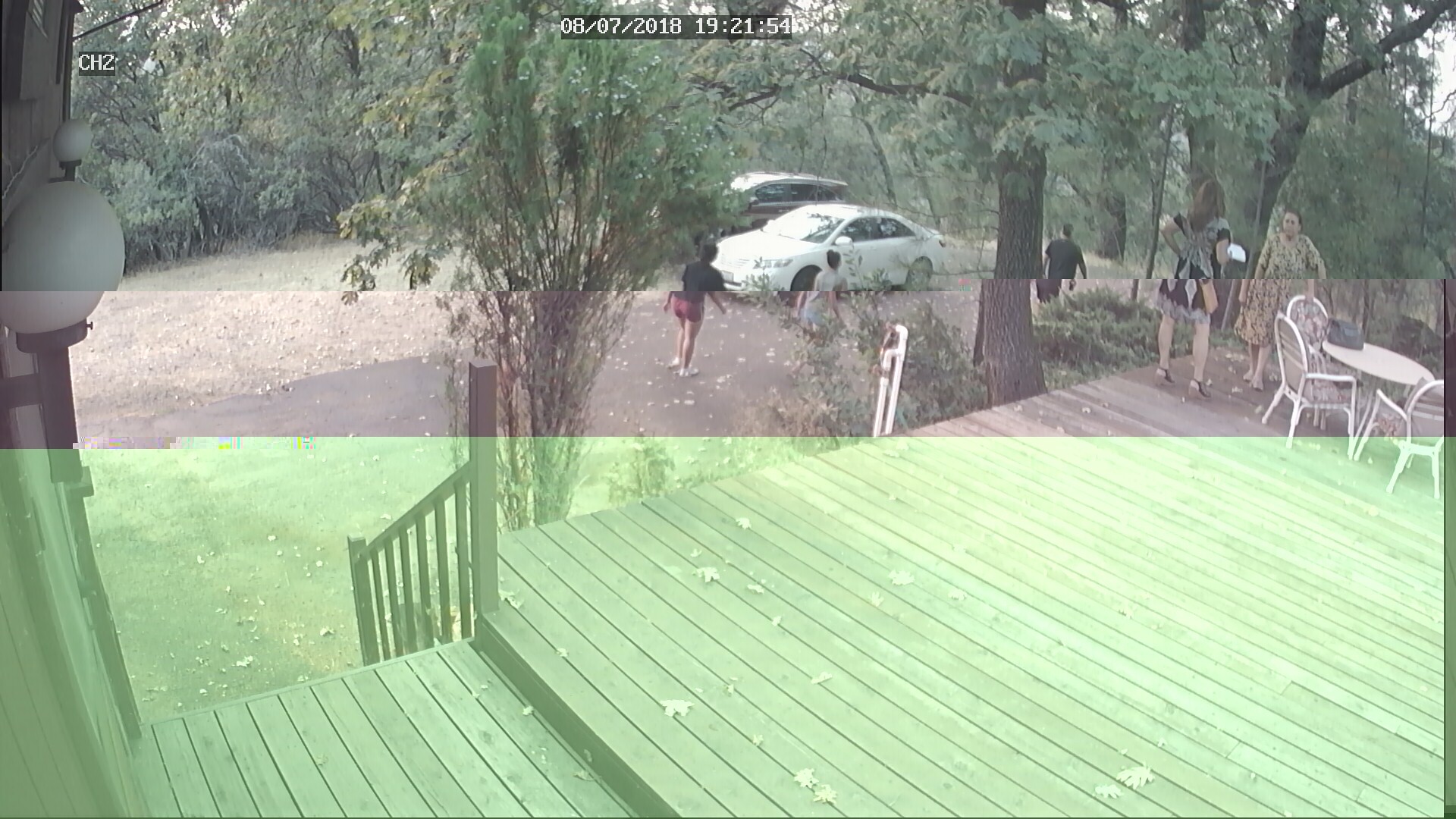This image, seemingly captured by a security camera, showcases an outdoor scene divided horizontally, with the lower half anomalously tinted in a translucent green, likely due to a camera malfunction. In the background, a group of people are gathered on a wooden deck—the deck itself a natural brown except for the distorted green section. 

To the right of the frame, there is a small metallic table accompanied by several chairs, around which two women are standing. One woman, sporting a short black hairstyle or possibly having her hair tied back, is dressed in a long green dress. The second woman, positioned to the left, is clad in shorts and a short-sleeved shirt patterned in black, pink, and gray.

Towards the center of the photograph, two vehicles are parked: a white car and a seemingly brown SUV. Near these vehicles, individuals are seen moving about. The leftmost person is dressed in a black short-sleeved shirt, red shorts, and white shoes. Beside this person is another individual with short black hair, wearing a gray shirt and possibly gray shorts.

Encircling the entire scene is lush greenery, with numerous trees and other vegetation suggesting a yard setting. The background also reveals a dirt driveway, reinforcing the impression of a private, possibly rural, location.